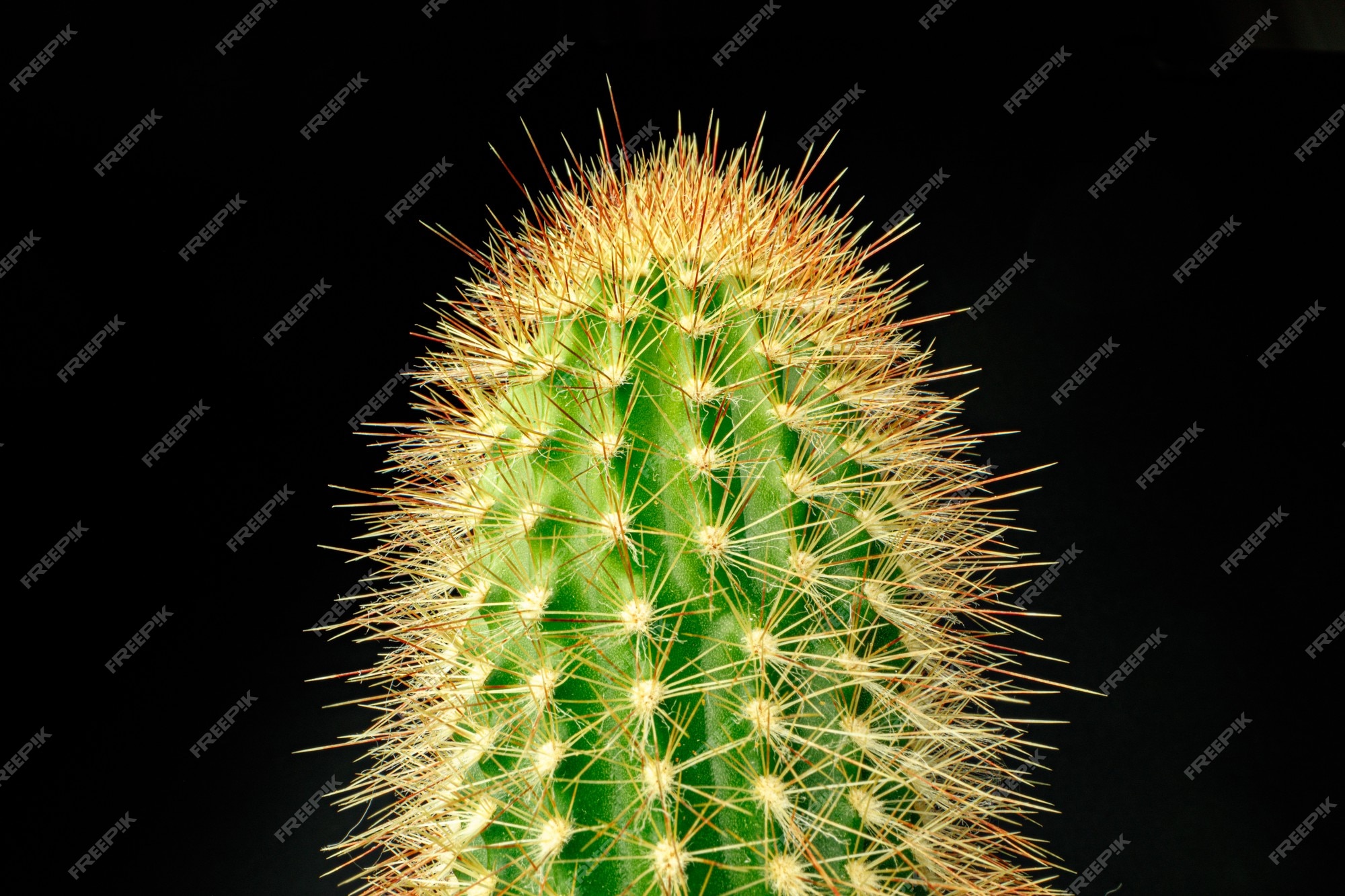In this image, a dome-shaped cactus head is prominently featured against a solid black background. The cactus is a vibrant green, with yellowish-white spikes emerging from its surface, their tips tinged in brown. These spikes are densely distributed across the top portion of the cactus. Surrounding this central figure, faint white text appears repeatedly in a diagonal pattern, forming the words "free pik," with "pik" spelled as P-I-K. The repeated text creates a subtle but intriguing backdrop to the strikingly detailed cactus.